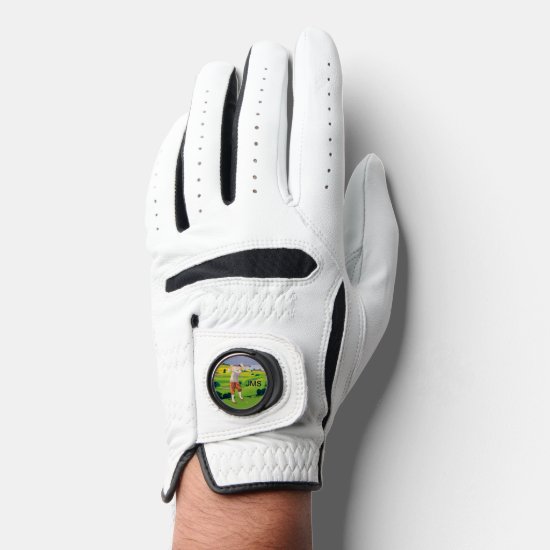This is a detailed top-down photograph of a person's hand adorned with a predominantly white golf glove featuring various design accents. The photograph shows a right hand with a fair complexion and some hair visible on the exposed wrist area extending out from the glove. The glove itself appears to be made of a plastic fiber rather than traditional leather. It has black detailing on the fingers (except the thumb), highlighted with ventilation holes in the white material on the top of each finger. The surface beneath the hand is completely white, though its nature—whether a table, shelf, or picture—is unspecified.

There are small grey dots forming a pattern on the top of the fingers for additional design and ventilation. The glove includes two noticeable black areas: one running horizontally across the glove and another vertically. Around the wrist area, the glove has an adjustable strap with a circular plastic decal featuring a cartoon image of a golfer in a light-colored shirt, red pants, displayed against a backdrop of green grass and a blue sky. The golfer is mid-swing with their golf club in the air, and the initials "JMS" are printed to the right of the image. The glove looks pristine, suggesting it hasn't been used in play, and the wrist area might include some elastic for a snug fit.